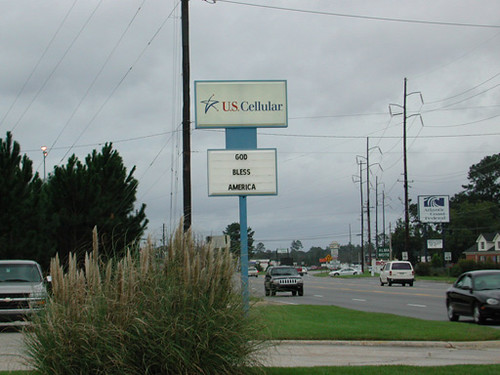This photograph captures a bustling street scene in America, centered around a prominent U.S. Cellular sign. The sign is held aloft by a light blue pole and consists of two main rectangular sections with a smaller blue rectangle separating them. The upper rectangle features a white background with a blue border, displaying "U.S. Cellular" in red and blue letters, accompanied by a blue star on the left. Below it, a message reads "God bless America" in black letters on a white background.

To the left of the sign is a large bush and a glimpse of a truck parked nearby, with some tall trees standing in the background. A four-lane road runs to the right, with several cars traveling in both directions. Electrical poles and power lines line the street, stretching off into the cloudy, overcast sky that suggests impending rain. The scene also includes a patch of pampas grass in the foreground and a vehicle situated in a parking lot area to the left of the image.